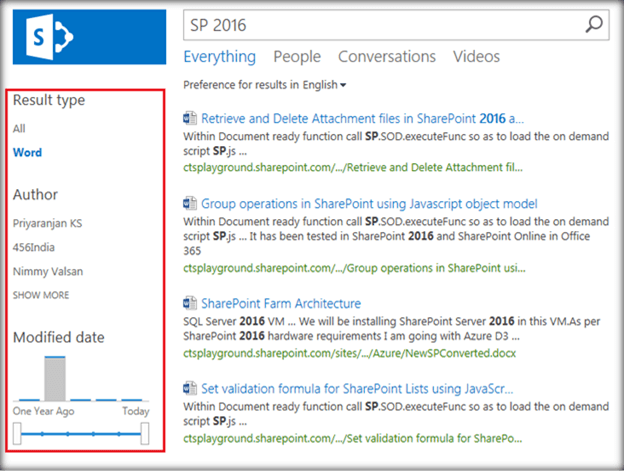In the upper left corner of the image, there is a blue rectangle containing an 'S' on a square, alongside a circle featuring three smaller circles. The 'S' is also blue. Adjacent to this, a search bar displays the text "SP 2016" followed by categories such as "everything," "people," "conversations," and "videos," with "everything" highlighted in blue while the others are in gray. Below the search bar, an option reads "preferences for results in English."

On the left side, there is a section titled "results type" with various options listed beneath it: "all," "word," "authors," followed by "PRIYARANJAN," "KS," "456," "India," "NIMI," "VASLAN," "VASLAN (V.A.L.S.A.N)," and a "show more" option. The modified date is noted as "one year ago today" and this section is encapsulated within a red rectangle.

Under the "everything" page heading, various blue hyperlinks are listed, including "Retrieve and delete attachment files in SharePoint 2016," "Group operations in SharePoint using JavaScript object model," "SharePoint farm architecture," and "Set validation formula for SharePoint lists using JavaScript." Each hyperlink is accompanied by a green URL.